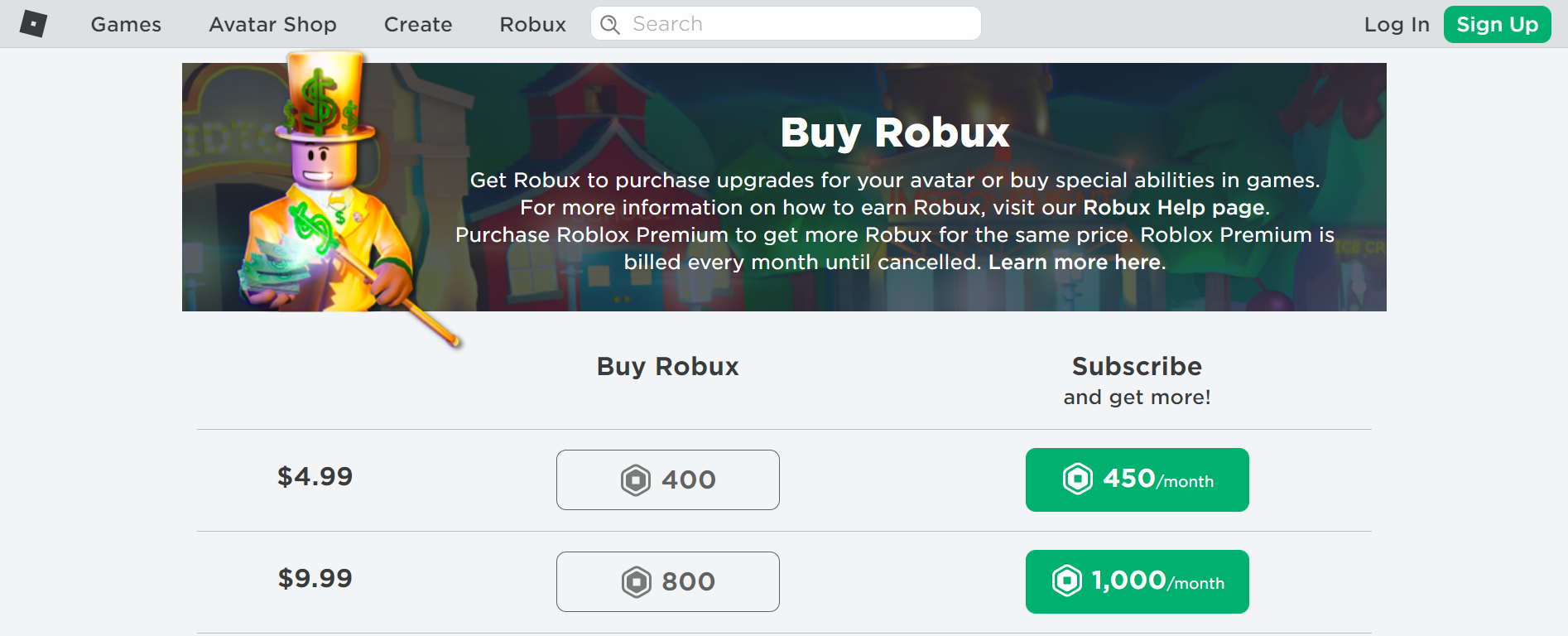The image depicts a webpage dedicated to purchasing Roblox in-game currency and subscriptions. The header of the website includes several navigation options on the top left: "Games," "Avatar Shop," "Create," and "Roblox." Adjacent to these, there is a white search bar for users to find specific items or information. On the top right, there are buttons for "Login" and a green "Sign Up" button.

Below the header, the main content area of the page introduces options to buy Roblox, upgrade avatars, and purchase special abilities within games. The text highlights that users can visit the Roblox help page for more information on earning Roblox, and encourages purchasing Roblox Premium for additional benefits. A note explains that Roblox Premium is billed monthly until cancelled, with a link provided for further details.

The background features a game-themed design with a prominent character on the left side. This character, styled like a Lego figure, is dressed in a gold suit and wields a gold stick with a green dollar sign, animatedly spawning money from his hand.

Underneath this banner, there is information about buying Roblox currency and subscription options. The text states, "Buy Roblox. Subscribe and get more." It specifies that for $4.99, users can receive 400 Robux or 450 Robux per month if subscribed, and for $9.99, they receive 800 Robux or 1,000 per month through a subscription. Both options are accompanied by green buttons.

The main content area has a grey background, providing a neutral backdrop for the information presented.